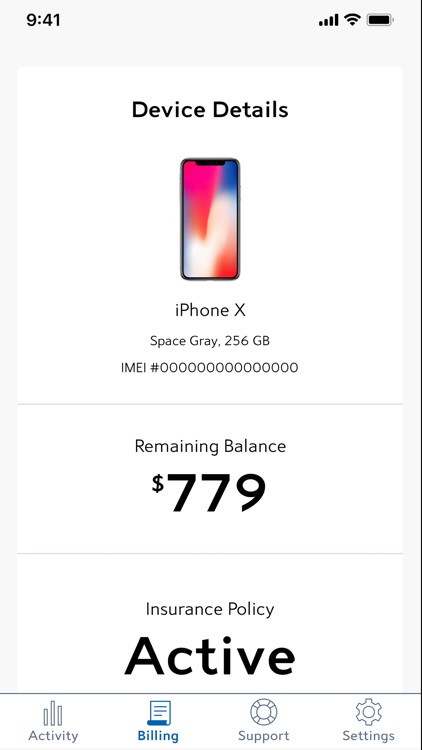The top portion of the image has a gray background showing standard smartphone status icons: the time "9:41," four signal bars, a Wi-Fi symbol, and a full battery indicator. Below this, the background turns white with the header "Device Details" in bold black text. 

The central portion displays a smartphone with a complex design featuring hues of purple, blue, red, and white, labeled "iPhone X" in Space Gray with 256 GB of storage. Just below this is the IMEI number, represented by a string of zeros.

Beneath these details, a horizontal line separates the information, followed by a "Remaining Balance" label. In large, bold black letters, it reads "$779."

Further down, another line separates the financial information from the insurance status, which shows "Insurance Policy" in bold black letters, marked as "Active."

At the bottom of the image, four buttons are aligned from left to right: "Activity," "Billing," "Support," and "Settings."